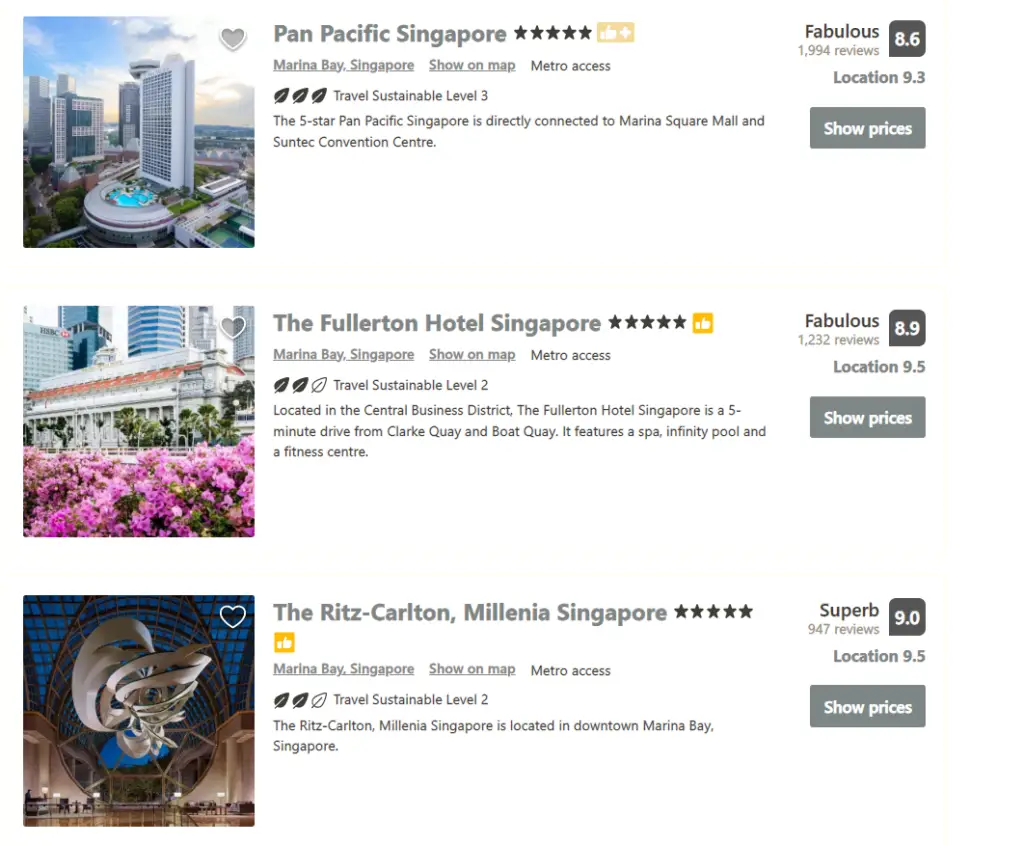This webpage features detailed information and rankings for three luxurious 5-star hotels in Singapore:

1. **Pan Pacific Singapore**
   - **Rating:** 8.6 (Fabulous)
   - **Location Rating:** 9.3
   - **Description:** The Pan Pacific Singapore offers contemporary, modern high-rise buildings with a large pool featuring a half-moon-shaped design around it. It boasts direct connectivity to the Marina Square Mall and Suntec Convention and Exhibition Centre, enhancing its appeal for both leisure and business travelers. The grey bar on the site indicates the pricing for accommodations.

2. **The Fullerton Hotel Singapore**
   - **Rating:** 8.9 (Fabulous)
   - **Location Rating:** 9.5
   - **Description:** Located in the Central Business District, The Fullerton Hotel Singapore provides a luxurious experience with a 5-star rating. It is situated just a 5-minute drive from Clarke Quay and Boat Quay. The hotel features a spa, an infinity pool, and a fitness center. It showcases an elegant blend of pink flowers and images of high-rise apartments, complemented by a low building accented with orange at the top. The prices can be checked through the grey bar on the page.

3. **The Ritz-Carlton, Millenia Singapore**
   - **Rating:** 9.0
   - **Location Rating:** 9.5
   - **Description:** This 5-star establishment is known for its modern design, highlighted by a striking statue in front of the building. Located in a prime area with a high location rating, The Ritz-Carlton, Millenia Singapore stands out for its sophisticated architecture and exceptional amenities. Pricing information is available through the grey bar featured on the website.

Each hotel provides a superb combination of luxury, convenience, and top-tier services, making them ideal choices for visitors to Singapore.